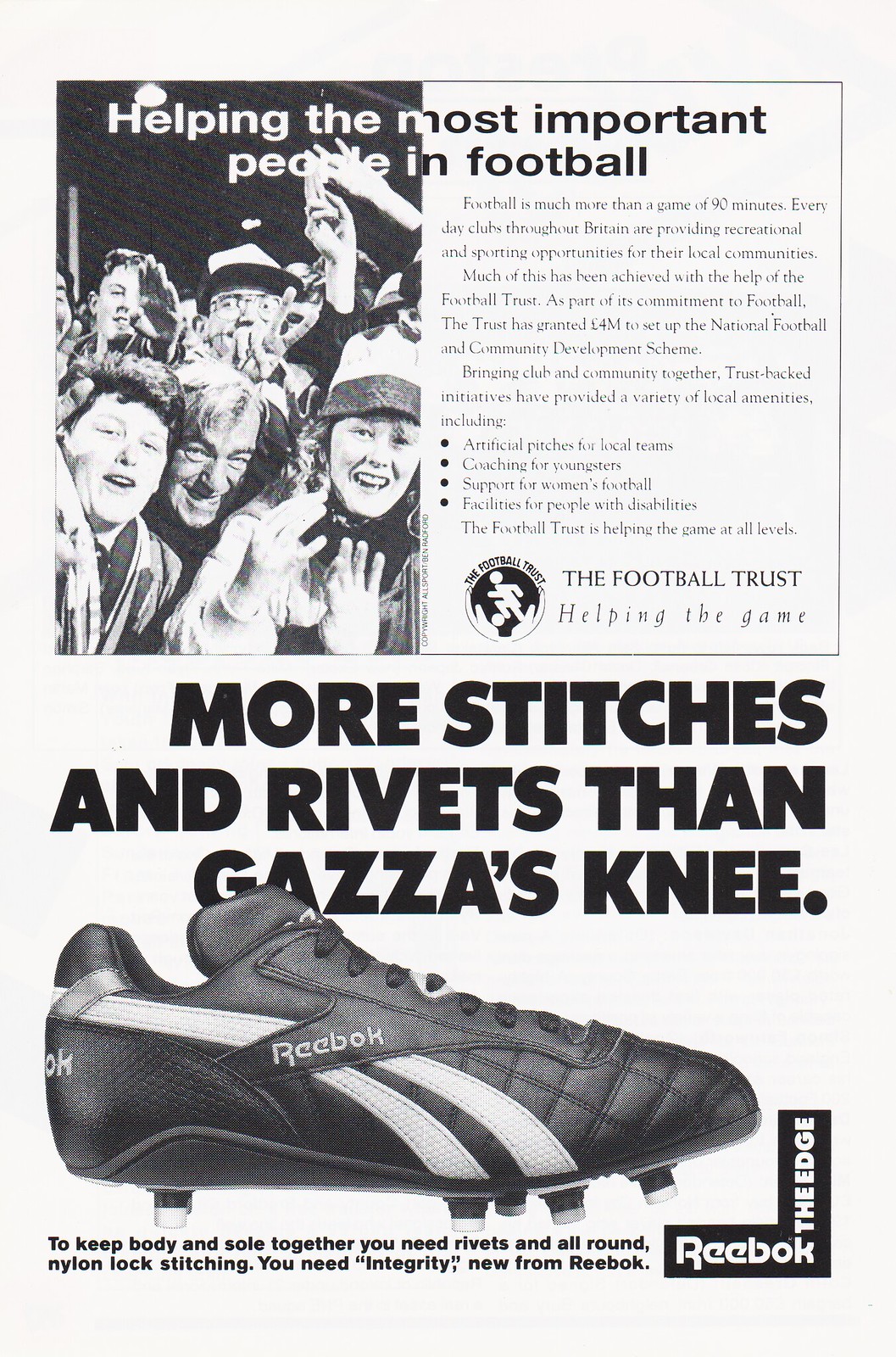This black-and-white magazine page features an older Reebok advertisement prominently. The top half showcases an ad for the Football Trust, with a headline that reads, "Helping the Most Important People in Football." An article discussing the significance of football in Britain accompanies the headline. On the left, a black-and-white photograph captures joyous soccer fans waving at the camera, illustrating a diverse crowd consisting of young, old, male, and female supporters. On the right, there's a logo of an animated soccer player within a circle, accompanied by the text, "The Football Trust Helping the Game."

The bottom half of the page is an advertisement for Reebok. Large, bold black letters declare, "More Stitches and Rivets than Gazza's Knee," referencing the famous soccer player Paul Gascoigne. Below this, a detailed black-and-white image of a Reebok cleat is displayed, showcasing the shoe's spikes designed for athletic use. The accompanying text beneath the shoe reads, "To keep body and soul together, you need rivets and all-round nylon lock stitching. You need Integrity. New from Reebok." This is followed by the iconic Reebok logo, completing the nostalgic sports advertisement.